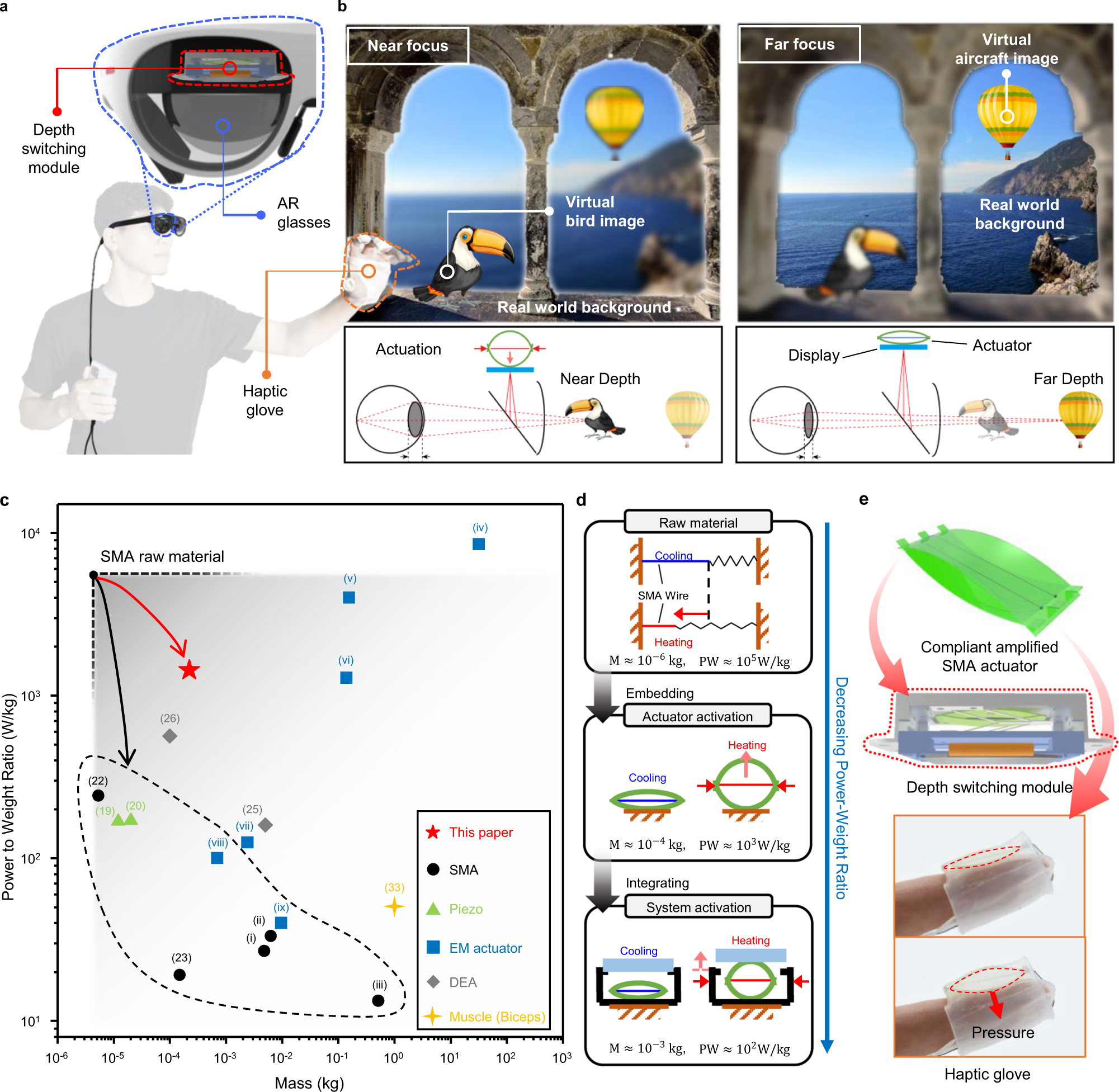The image depicts a comprehensive diagram illustrating the functionalities and components of an AR system, focusing on AR glasses and a haptic glove. In the top left corner, there is a faded image of a boy wearing these AR glasses, which are labeled "Depth Switching Module," and a haptic glove on his left hand. The images to the right detail the operational capabilities of the glasses: 

- Part A introduces the system with a boy wearing the AR glasses and haptic glove.
- Part B shows two diagrams of an outdoor scene viewed through the AR glasses. The first image, labeled "Near Focus," presents a clearly visible virtual bird labeled "Virtual Bird Image" with a blurred background, while the second image, labeled "Far Focus," shows the same scene with the background clear and a hot air balloon labeled "Virtual Aircraft Image" with the bird blurred out. This demonstrates the depth-switching capability of the glasses, controlled by an actuator that shifts the display to adjust depth of field.
- Part C contains technical graphs and mathematical formulas, illustrating a power-to-weight ratio versus mass and details on the raw material's performance over time, which are likely related to the AR system's components but are not directly explained.
- Part D focuses on the haptic glove, showcasing an actuator on the fingertip and indicating a pressure mechanism in kilograms, emphasizing how the glove interacts with the virtual environment via tactile feedback.

Overall, the diagram thoroughly explains the integration and function of AR glasses and a haptic glove, highlighting their depth-switching technology and haptic interaction capabilities.